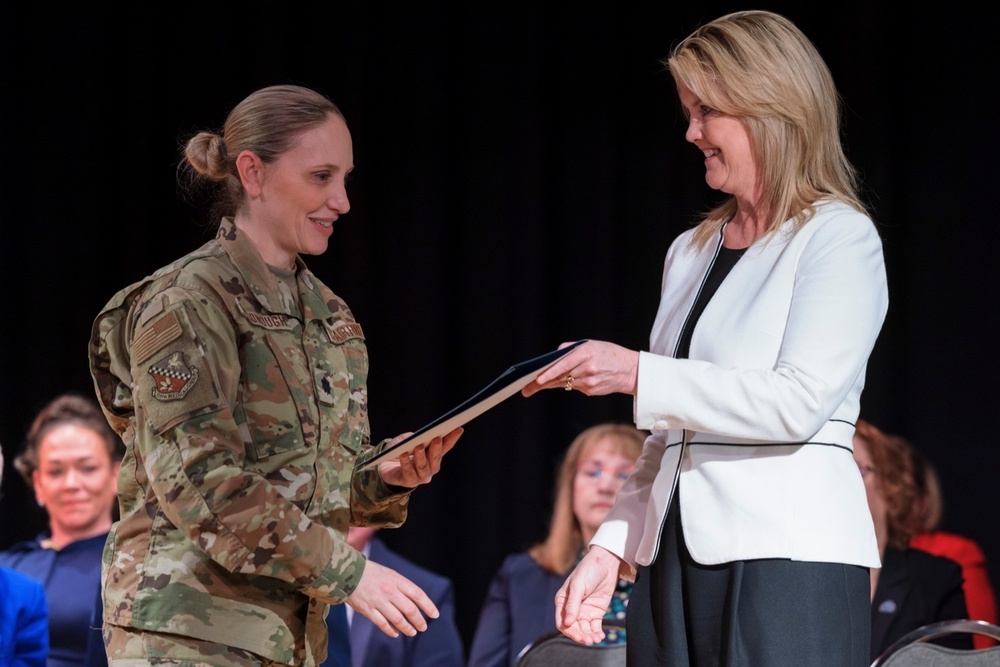In this professionally composed photograph, set against a black backdrop, a smiling female U.S. Army soldier in green camouflage fatigues, with a neatly pulled-back bun, stands to the left. The U.S. flag is visible on her uniform sleeve. She is gracefully accepting an award from another woman on the right, who is impeccably dressed in a white blazer and black pants. This woman, with straight blonde hair, looks down as she hands the award to the soldier. The event appears ceremonial and dignified, possibly a graduation or recognition ceremony, evidenced by several attendees sitting behind them, wearing formal robes, and smiling. The image, wider than it is tall, tastefully centers the focused interaction, capturing a moment of honor and achievement.